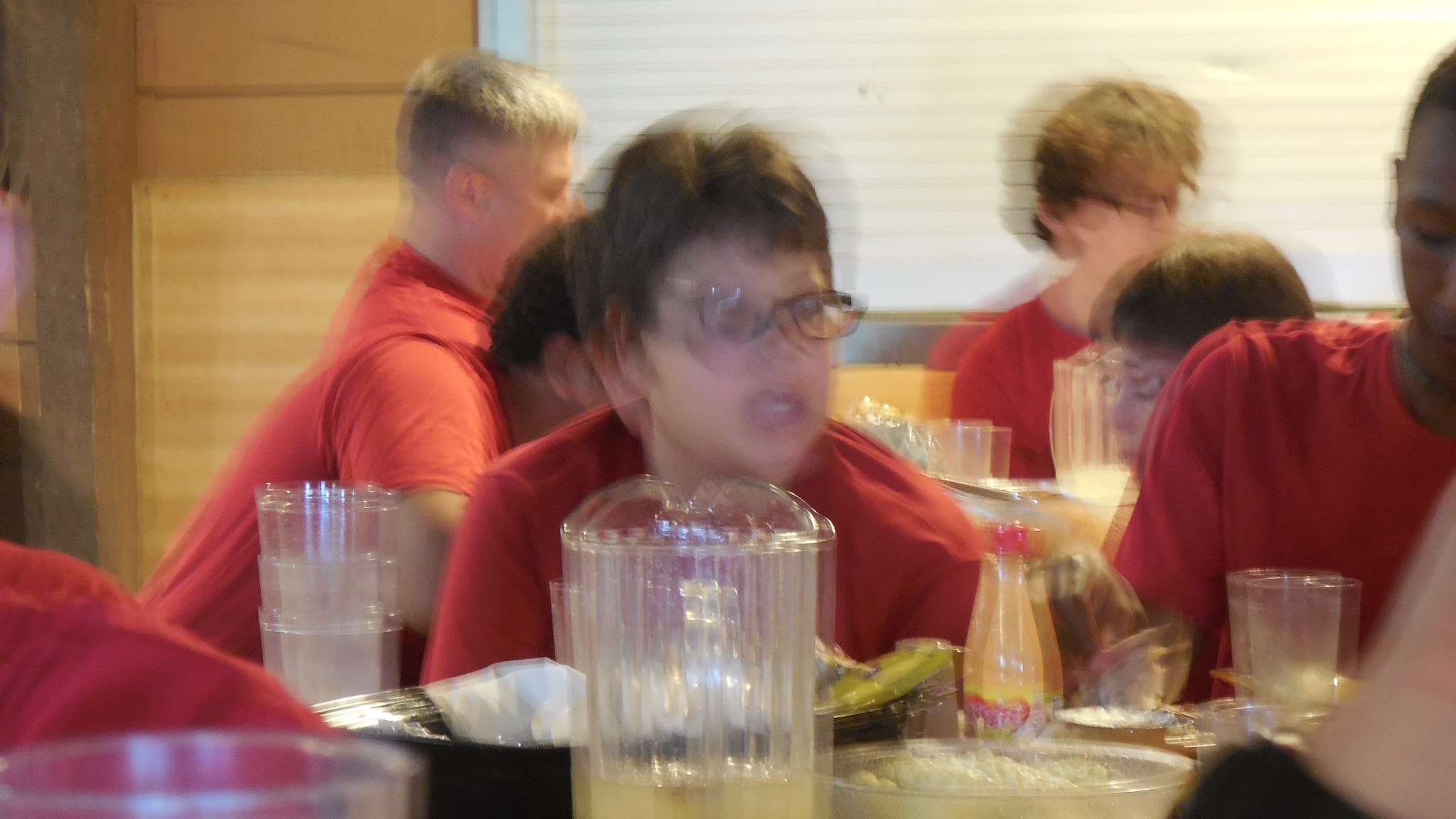In a very blurry and out-of-focus photograph, a group of young boys, all approximately under 15, are captured sitting in what appears to be a summer camp dining room. They're wearing identical red t-shirts, suggesting a uniform or a common event. The scene shows several long, bench-style tables with clear plastic water pitchers and plastic cups arranged on them. The most prominent boy in the foreground, a white boy with messy brown hair and black glasses, has a noticeably blurred face as if he was in motion. Beside him, to his left, is a young black boy also in a red shirt. Scattered across the tables are plates, empty glasses, and in one instance, a bottle of juice. Behind the main table, another table is visible with at least three boys, and further back, two older white adults with glasses and another young boy, all in red shirts. The background reveals a big window with blinds and light wood grain walls, hinting at a casual and cozy camp dining hall environment.